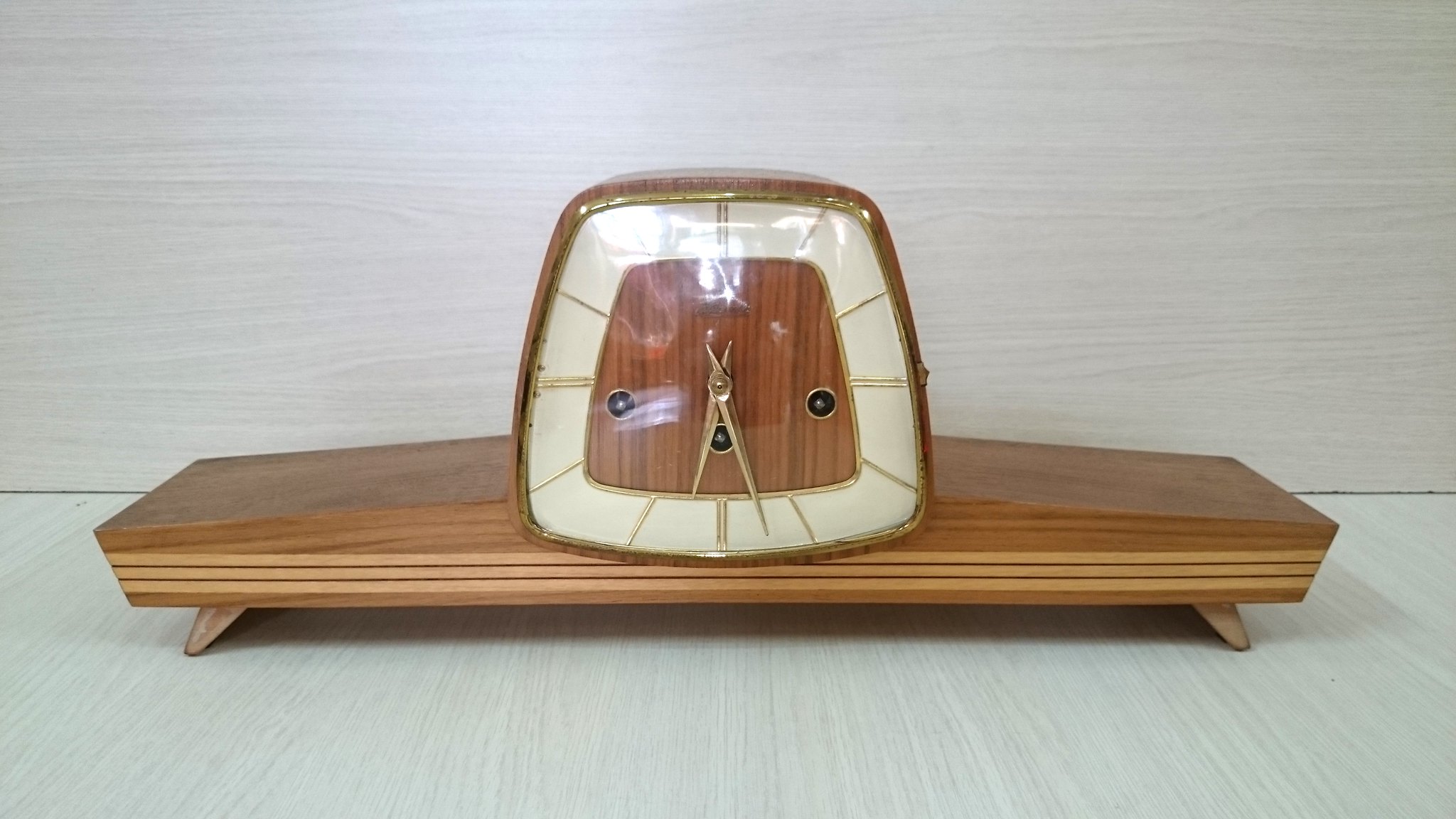This landscape-oriented photograph features an antique clock prominently displayed on a wide, low-standing base. The base, made of wood with a matching grain pattern, spans approximately three times the width of the uniquely shaped clock face. The clock itself has no numerical digits, displaying only gold-colored hour markers. The hour and minute hands, also gold-colored, indicate the time as approximately 5:27. The clock's background is a rich, wooden texture, consistent with the stand it rests on. Both the clock and its stand are placed on a surface adorned with a light gray striped pattern, adding a subtle contrast to the warm wood tones of the timepiece.